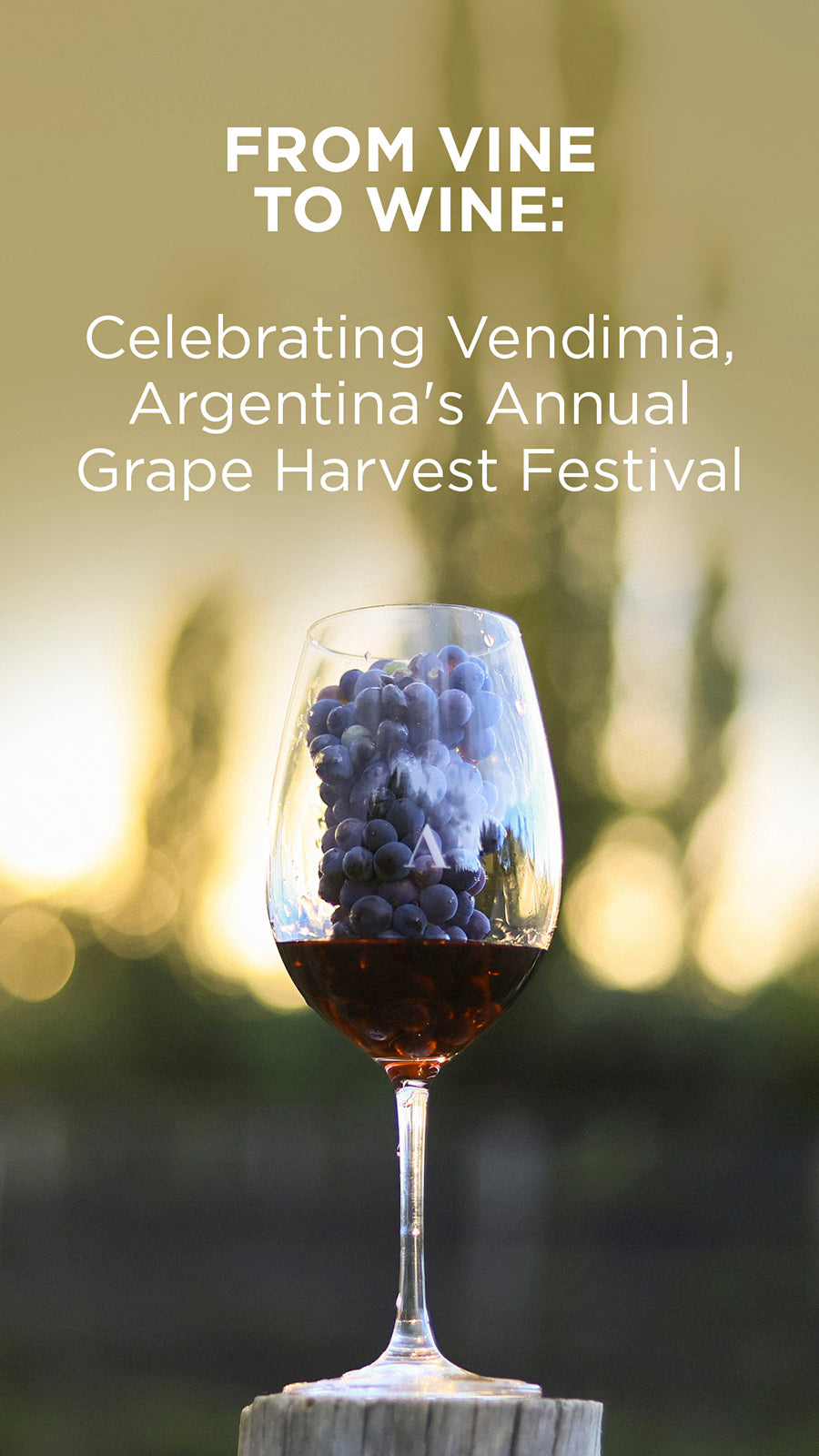This image is a detailed advertisement for a wine festival. At the top, set against a grayish-brown background, white letters announce "From Vine to Wine: Celebrating Vendemia, Argentina's Annual Grape Harvest Festival." Below this heading, a wine glass, partially filled with red wine, prominently features a cluster of purple grapes. The wine glass, balanced on a piece of wood, is set before a blurred backdrop featuring hints of lights, trees, and a golden sunset that casts a yellowish hue, evoking an outdoor scene at golden hour.